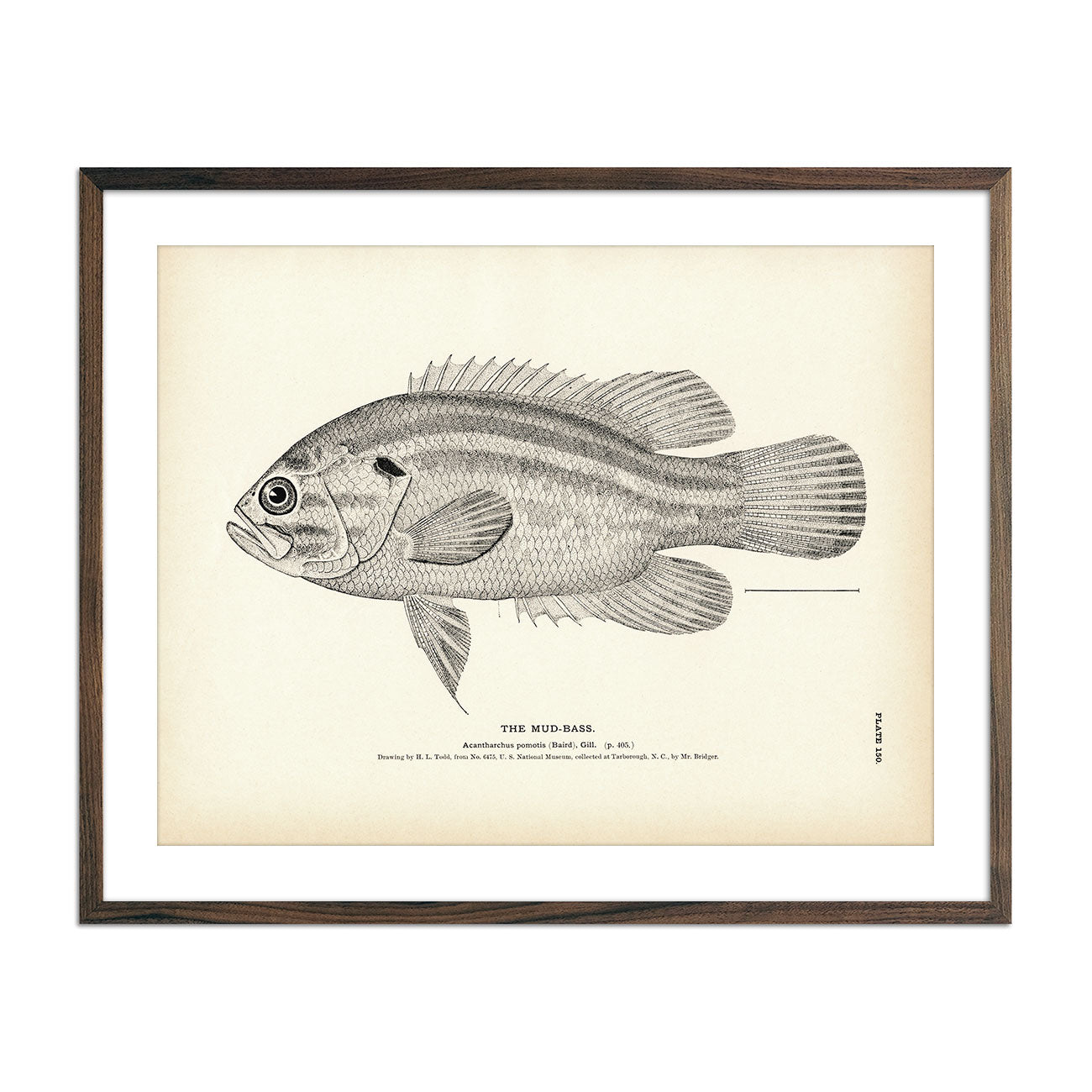The image features a highly detailed, black-and-white pencil drawing of a fish, specifically the Mud Bass (Acantharchus pomotis). Encased in a thin brown wooden frame with white matting, the drawing is rendered on light brown paper. The fish is depicted in profile, with its face oriented to the left, displaying one visible eye and a slightly open mouth. The intricate scales and the two distinct gray stripes running the length of its body are meticulously shaded. The Mud Bass is illustrated with spiny fins on both its top and bottom, a smooth tail, and side fins. Text at the bottom of the image includes its Latin name, "Acantharchus pomotis," with additional details such as "Baird and Gill, P405," and credits the artist H.L. Todd, along with the collection location, Turborough, North Carolina, by Mr. Bridges. A measurement scale is present along the side, although the numbers are not legible. The drawing is identified as "Plate 150," which is indicated by vertically aligned text on the right side.